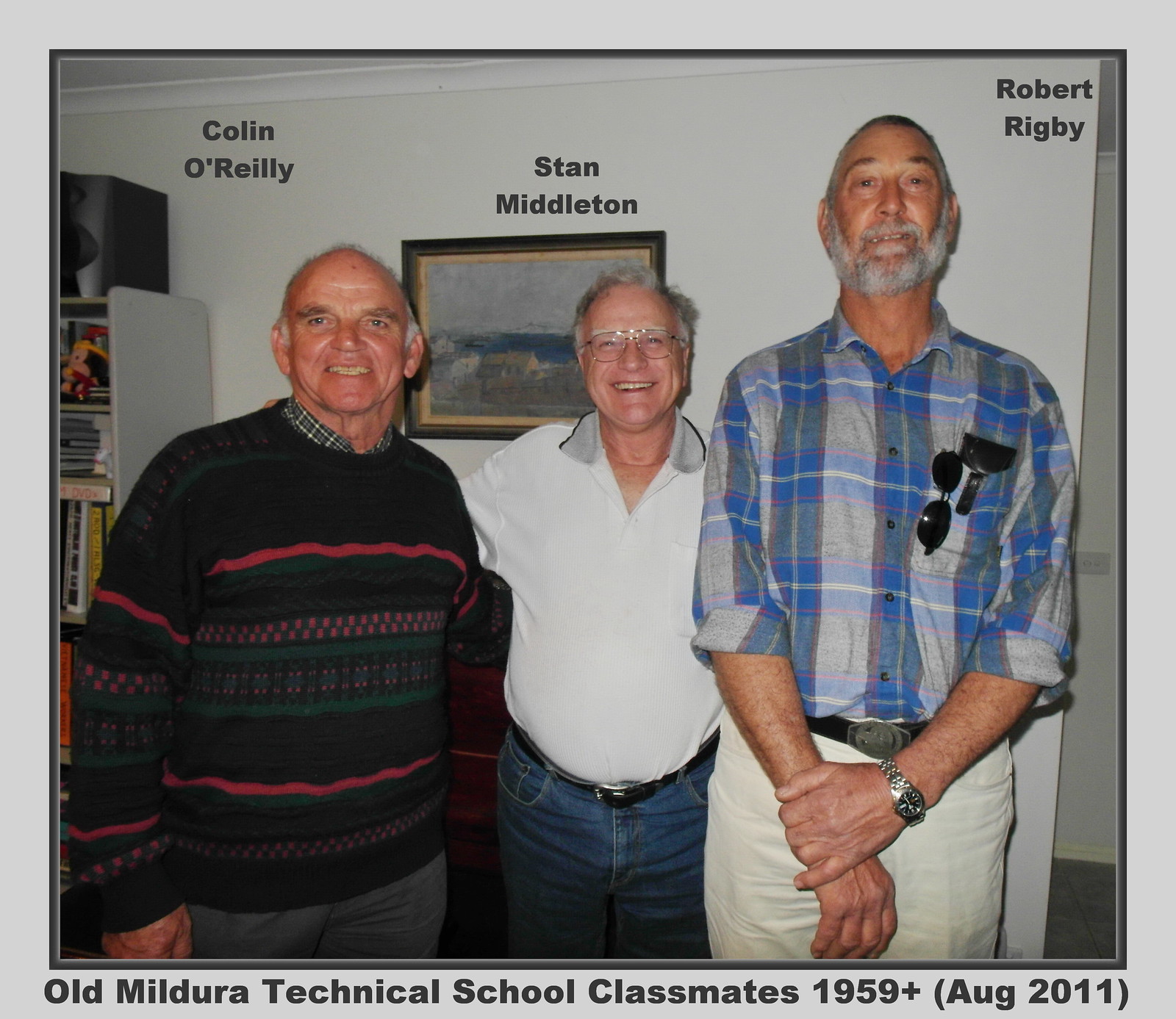In the photograph, three older men, identified as Colin O'Reilly, Stan Middleton, and Robert Rigby, are seen standing in a well-lit living room, with a white-painted background adorned by picture frames, bookshelves, and a distinctive Monet painting. Colin O'Reilly, positioned on the left, sports a black sweater with vibrant stripes of red, green, yellow, and blue, paired with gray pants. With his balding gray hair, Colin smiles warmly. In the center is Stan Middleton, distinguished by his white glasses and his arm around Colin. Stan wears a white polo shirt with a gray collar and blue jeans. Robert Rigby stands on the right, noticeably taller than his companions, donning a blue and gray plaid shirt with sleeves rolled up, light beige pants, a watch, and sunglasses peeking from a pocket. He also has a gray beard and hair. All three men, who are smiling, have their names written above their heads, and the caption at the bottom of the photograph reads, "Old Mildura Technical School Classmates, 1959+, August 2011," indicating their long-standing friendship since their school days and the date the photo was taken.